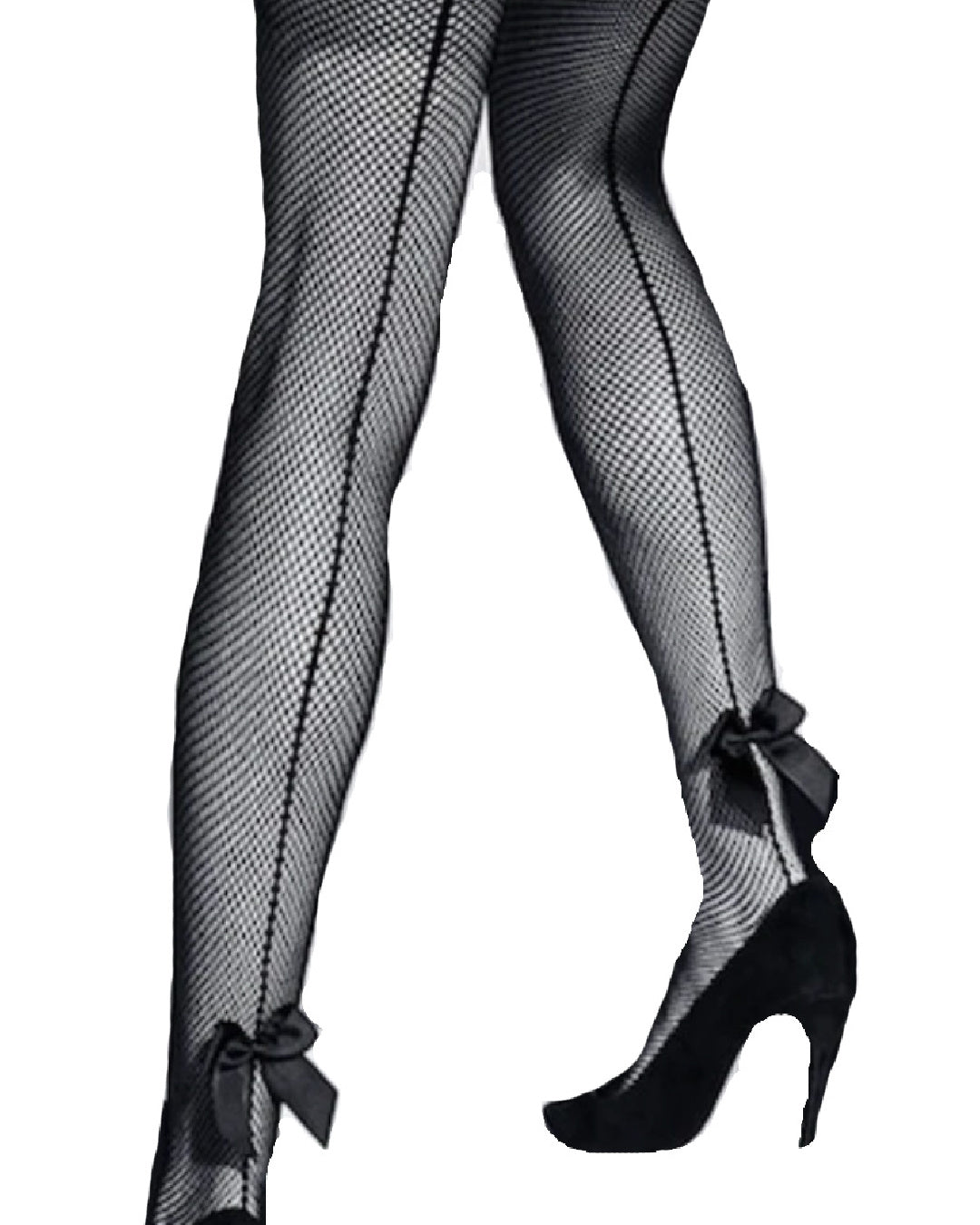This detailed black and white photograph captures the legs of a woman adorned in fishnet stockings, viewed from the rear. The image is cropped just above the upper back thigh, revealing only her calves, hamstrings, and the back of her upper thighs. Both legs are encased in fishnet stockings that extend down to high heels. On her left leg, positioned on the left side of the image, only the very top sliver of her high heel is visible. Both stockings feature a seam running down the back, adding a vintage allure to the ensemble.

A small, dark-colored ribbon adorns the base of each stocking, just above the high heels, which also appear very dark due to the monochrome nature of the photograph. The high heels themselves are striking, towering at an estimated height of at least five inches. The composition and intricate details create an evocative and stylish depiction, emphasizing the textures and patterns of the stockings and the elegance of the high heels.